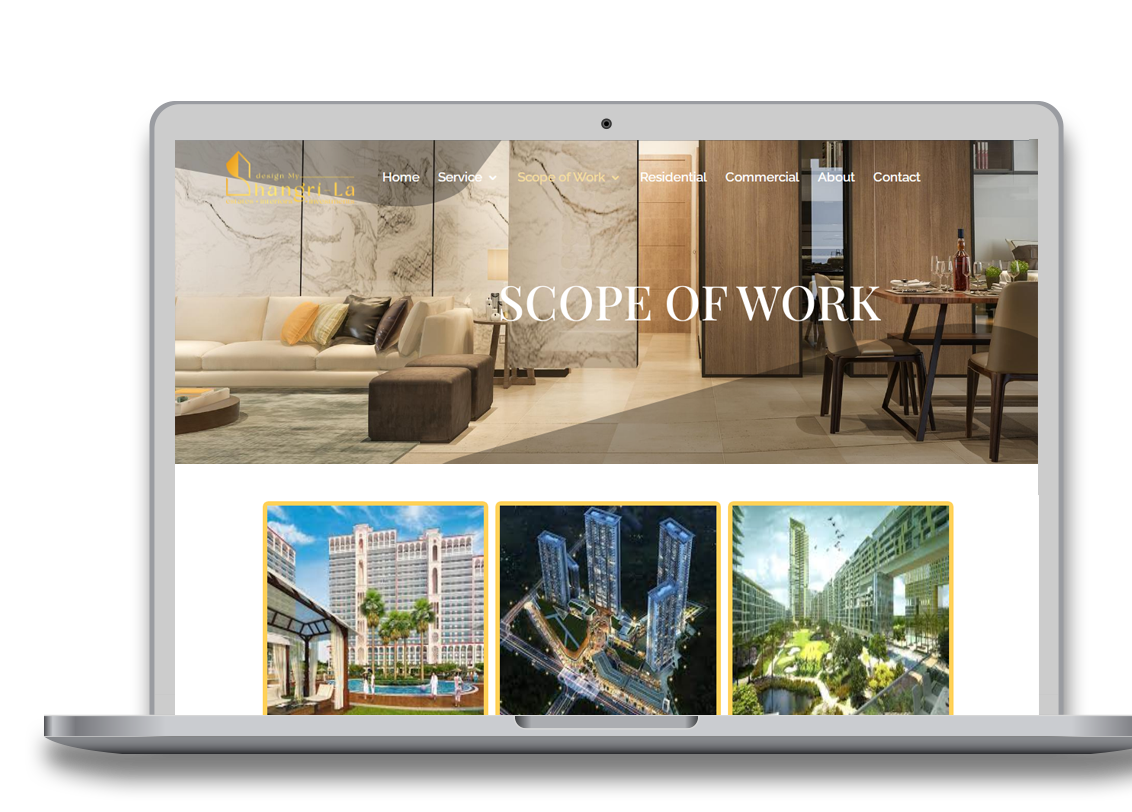A digitally rendered image of an open laptop is displayed. The laptop is showcased from the front edge of the keyboard, extending to an upright screen. The keyboard, touchpad, and base are meticulously detailed, capturing the essence of a modern device. The screen is active with a photo of a website.

The website's banner image depicts an elegant interior room. On the left side, there is a sofa adorned with five intricately designed throw pillows. To the right, a dining table is set, featuring a bottle of wine and several wine glasses. The top left of the banner bears the name "Shangri-La" alongside a yellow logo, both overlaying a marble-textured background, making the text somewhat challenging to discern.

Navigation options are arrayed at the top of the webpage: Home, Services (with a drop-down menu), Scope of Work (with a drop-down menu), Residential, Commercial, About, and Contact. Prominently in the center of the banner, "Scope of Work" is displayed in white text.

Below this broad photograph banner, the background transitions to white. Here, three square thumbnail images, each outlined in yellow, are strategically placed. The leftmost thumbnail features a grand hotel accompanied by a pool. The central image presents an impressive aerial view of four towering skyscrapers. The rightmost thumbnail appears to be an architect's rendering, illustrating a garden interspersed with high-rises.